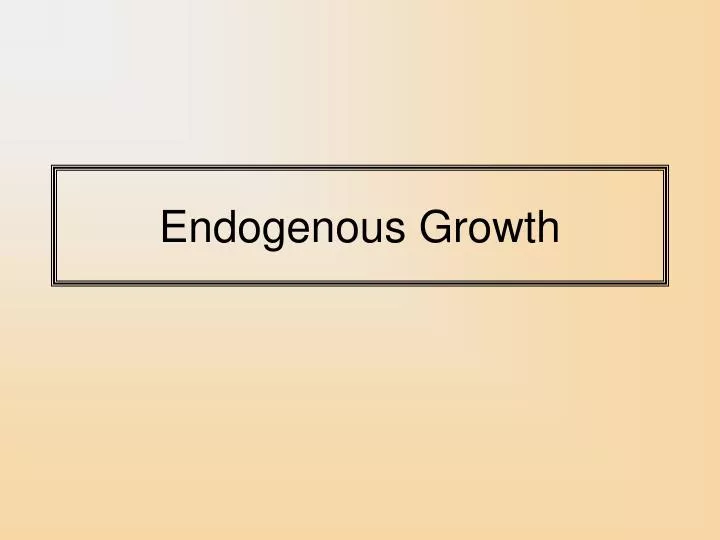The image features a peach-colored background that transitions into a very light blue or gray color in the upper left corner. Centered horizontally but slightly above the middle, there is a black-outlined rectangle with three lines: a thin outer line, a thicker middle line, and an inner thin line. Inside the black rectangle, the words "Endogenous Growth" are written in black letters, both words starting with capital letters. The text is centered within the rectangle, and the background within the rectangle matches the peachy tone of the overall background.